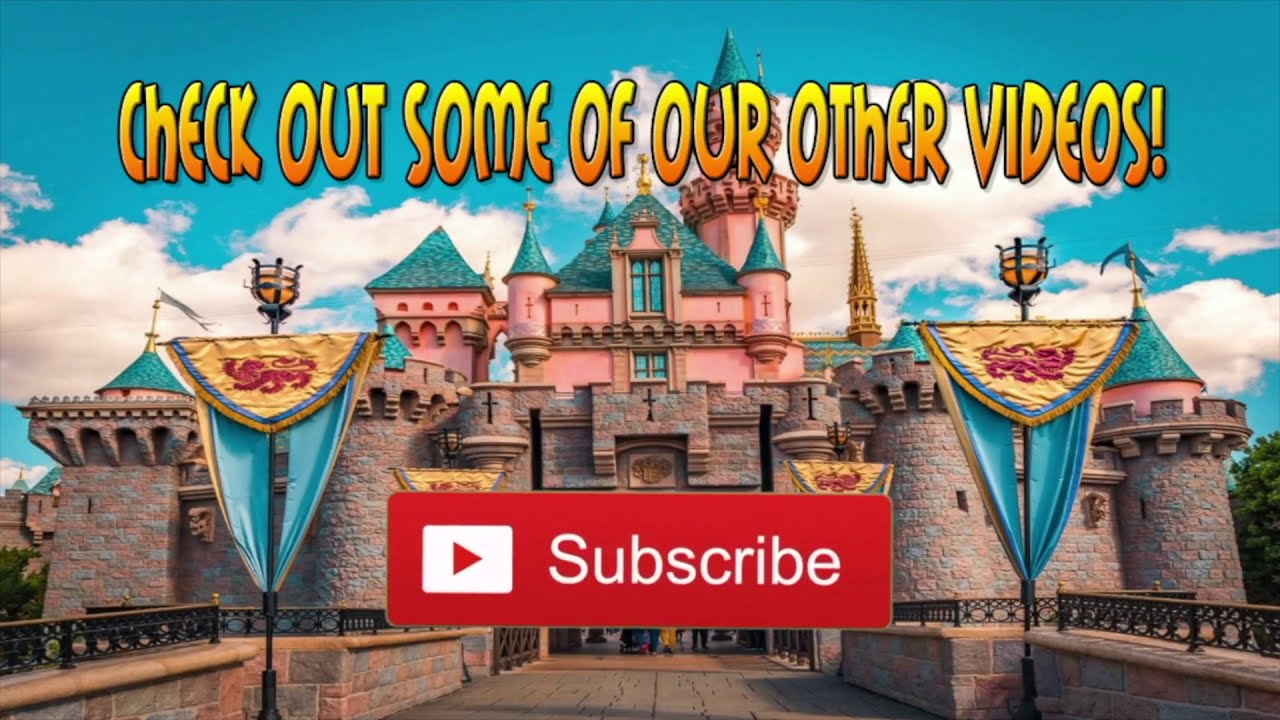This image showcases a detailed and colorful rendering of a grand castle, set against a vivid blue sky dotted with white clouds. The castle itself features a mix of stone-gray, pink, and blue hues. It boasts a towering structure with steeples and a green roof. The front castle wall is more muted, resembling traditional stonework, and partially obscures the taller, more vibrant pink sections of the castle behind it.

The entrance to the castle is adorned with massive stone columns and is framed by a bridge or wide walkway leading up to it. On either side of the entrance, there are two yellow lanterns accompanying flags in shades of gold, blue, and red, possibly displaying a lion design.

A red rectangular subscribe button with white lettering stretches across the bottom part of the image, covering the castle's large door. However, you can still see the feet of several people underneath this button, suggesting activity and movement toward the entrance. At the top of the picture, a yellow-orange text reads, "Check out some of our other videos."

In the background, to the right and left edges of the image, green trees can be spotted, along with another stone castle-like building on the left, adding more depth to the scene.